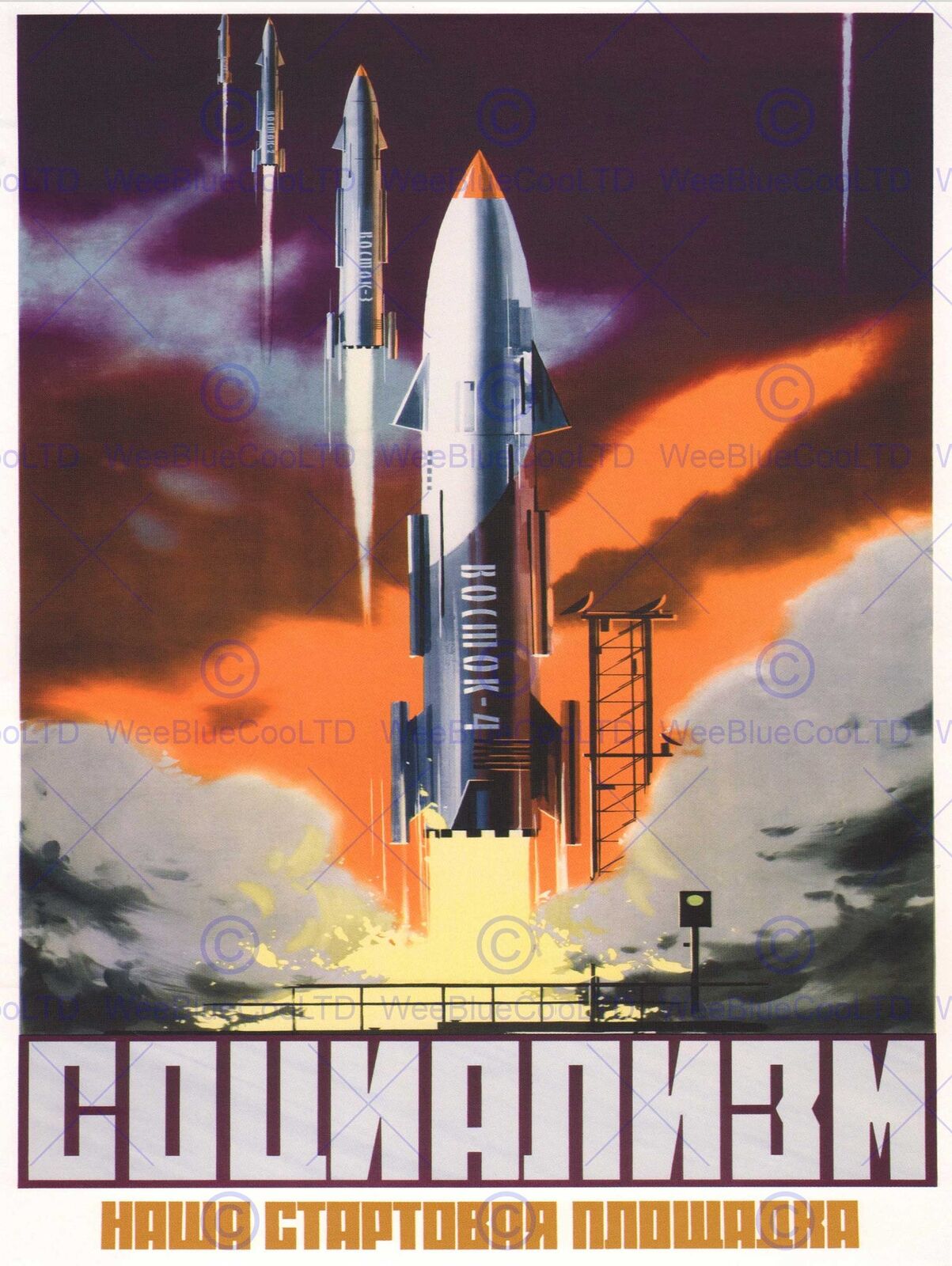The image is a modern-art-style graphic poster featuring a central rocket ship that's barely off the ground, emitting yellow lights and gray puffs of smoke from its base as it takes off. The rocket, slender with a light silver and dark gray body, has a red, almost triangular point at the top. The sky behind transitions from a dark purplish hue to a reddish-crimson tint, blending into an orange color. In the background, several smaller rockets ascend at various heights; one is situated just to the upper left of the main rocket with white smoke trailing, and another is even further back. The top right of the image features a tiny, distant rocket. The bottom of the poster contains text in a foreign language, possibly Russian or Eastern European, and there is a watermark stating "copyright, We Blue Cool LTD."